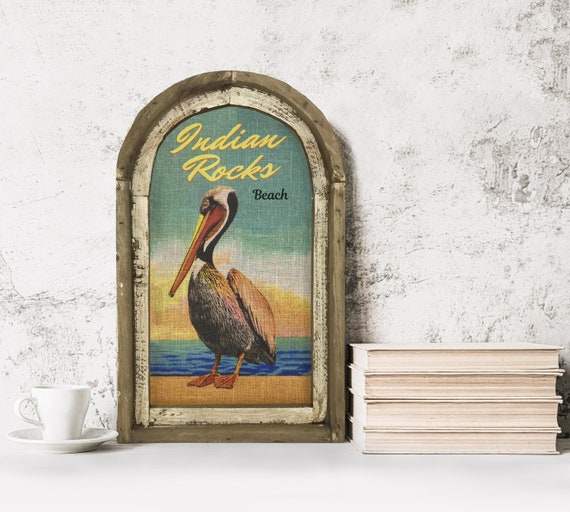The image depicts a framed print of a pelican standing on a beach with the ocean visible in the background, along with the text "Indian Rocks Beach" written in a yellow, semi-cursive font. The frame itself is dual-layered, with an inner light wood-colored mat and an outer darker wood layer, giving it an arch or doorway shape. The scene within the frame showcases a pelican with a black and white marked head and a brown body, set against a blue ocean with a yellow, white, and green sky, indicative of a tropical setting at sunset. The framed picture rests on a white table with a white and gray textured wall behind it. To the left of the frame is a white coffee cup and saucer, and to the right are four stacked ivory-colored books with their pages facing forward and spines against the wall.